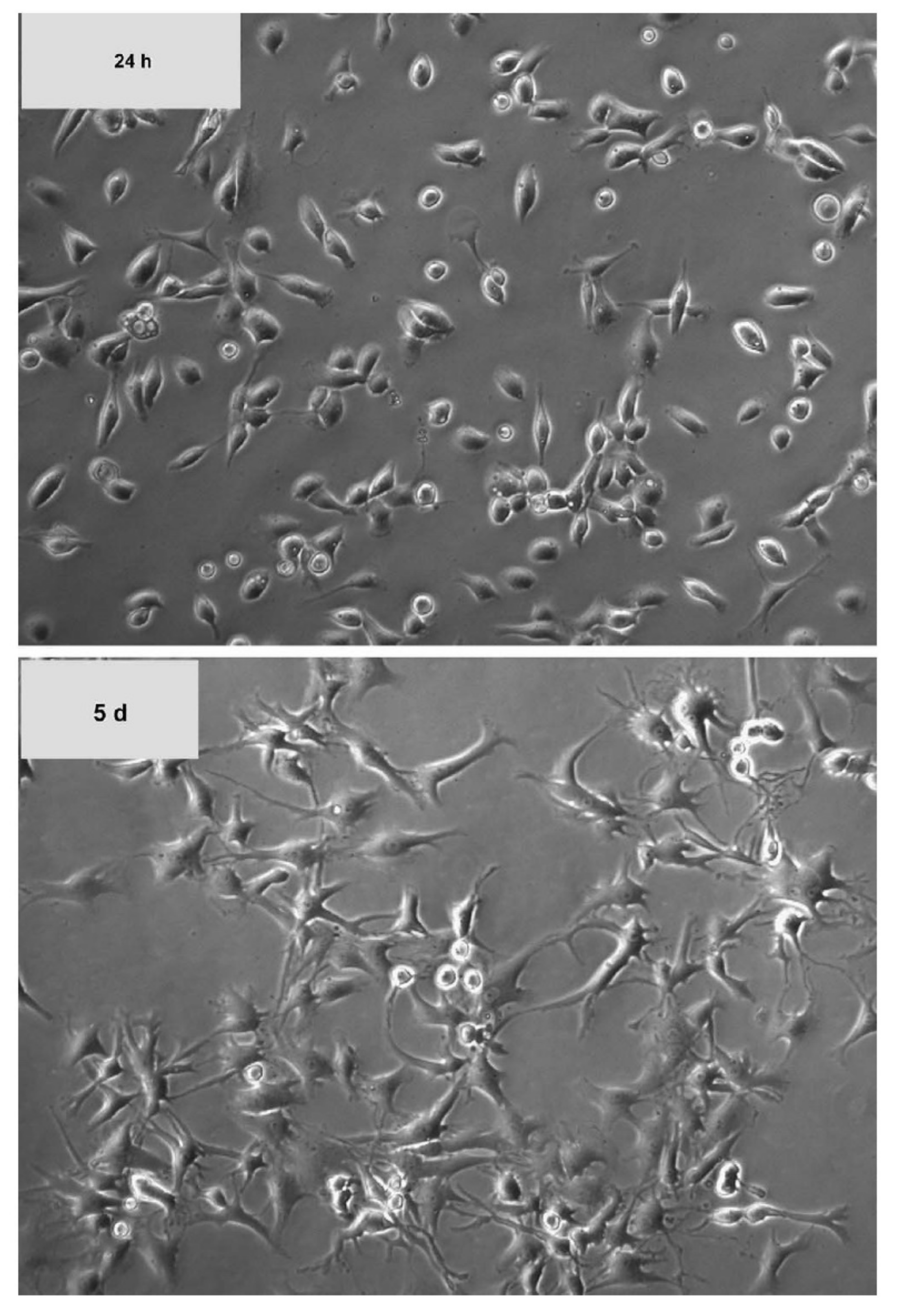This image displays two microscopic photographs, positioned one above the other, capturing the progressive growth of microorganisms over time. The top photograph is labeled "24 hours" and the bottom one "5 days." Both images feature a monochromatic palette of black, gray, and white. At the 24-hour mark, scattered microorganisms can be observed throughout the frame. By the 5-day mark, the number of microorganisms has notably increased, densely populating the visual field. The chronological comparison highlights the accelerated proliferation of these microorganisms over the extended period.